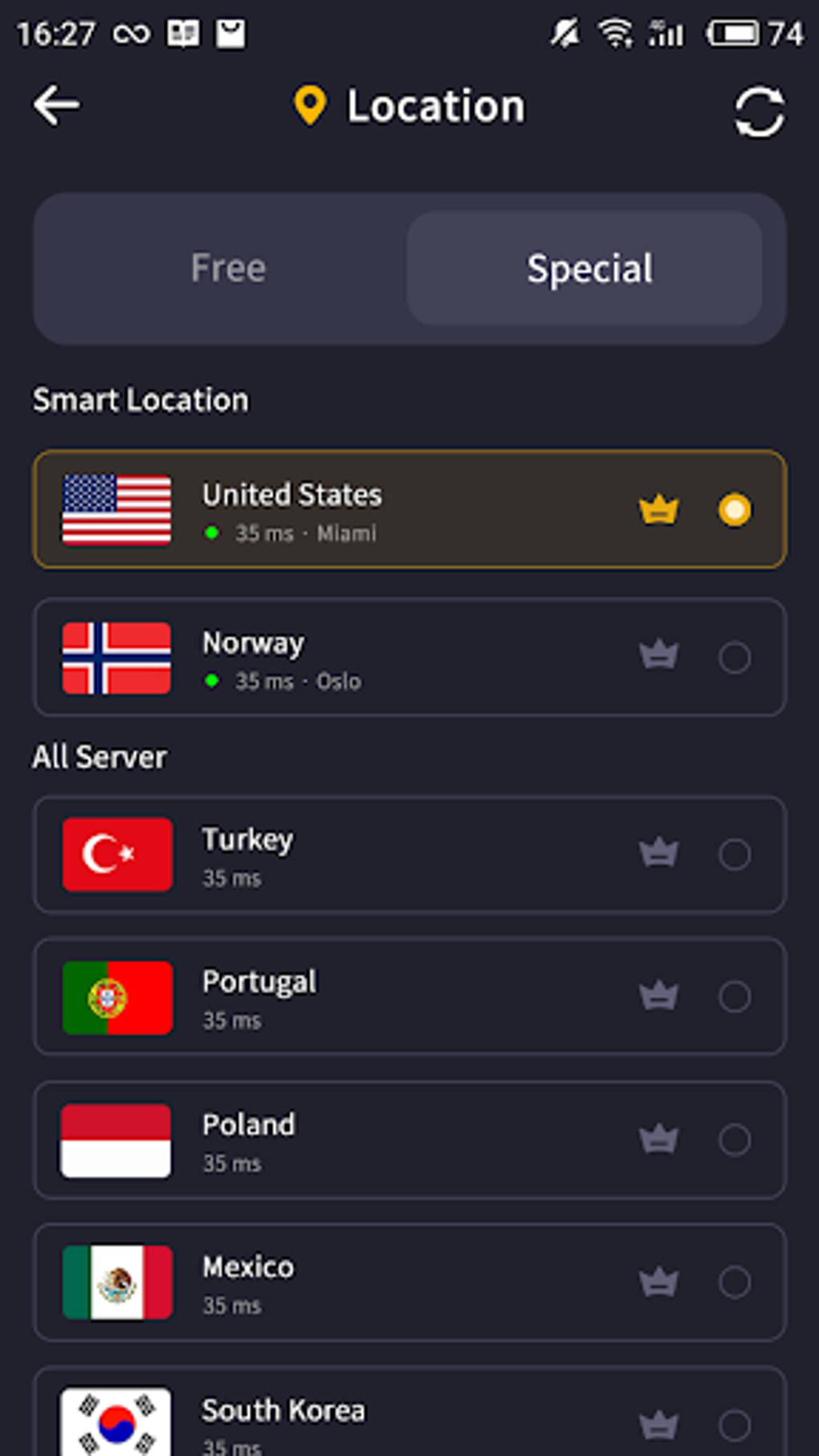**Screenshot Description**

The screenshot displays a mobile phone interface with the current time shown as 16:27. At the top of the screen, several icons are visible, including a battery level indicator at 74%, Wi-Fi signal, and either 4G or 5G network connectivity. There is a left-facing arrow in the top banner, next to the text "Location" accompanied by a location icon, and a refresh icon nearby.

Below the top banner, there are two buttons labeled "Free" and "Special," with the "Special" button currently highlighted. Under these buttons is a list of server locations presented with country flags. Each list item shows the country name, a flag, and server latency in milliseconds (MS):

1. **United States**: Flag of the United States, 35MS Miami (Highlighted with a green light)
2. **Norway**: Norwegian flag, 35MS Oslo (Highlighted with a green light)
3. **Turkey**: Turkish flag, 35MS
4. **Portugal**: Portuguese flag, 35MS
5. **Poland**: Polish flag, 35MS
6. **Mexico**: Mexican flag, 35MS
7. **South Korea**: South Korean flag, 35MS

These details provide an organized view of available server locations for a virtual private network (VPN) or similar application, with the United States and Norway being indicated as the preferred options based on their green lights.